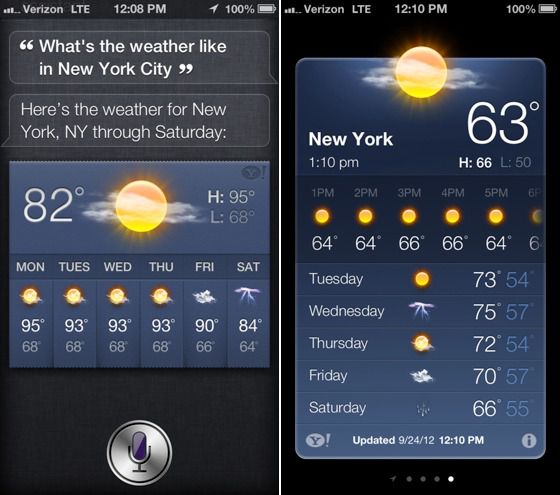Two side-by-side smartphone screenshots comparing weather forecasts for New York City. 

The left screenshot, taken at 12:08 PM with a 100% battery, features a black background and showcases an AI-assisted weather query. The screen displays the question, "What's the weather like in New York City?" with the AI's response, "Here's the weather for New York, New York through Saturday," followed by a seven-day forecast.

The right screenshot, captured at 12:10 PM, delves deeper into the weather details without AI assistance. It provides the same seven-day forecast along with an extensive hourly breakdown for the current day, displaying high and low temperatures for five full days. The additional information includes hourly temperature variations, offering a more comprehensive view of the weather conditions.

This visual comparison highlights not only the time difference and battery life but also the varying levels of detail accessible through different methods of checking the weather.